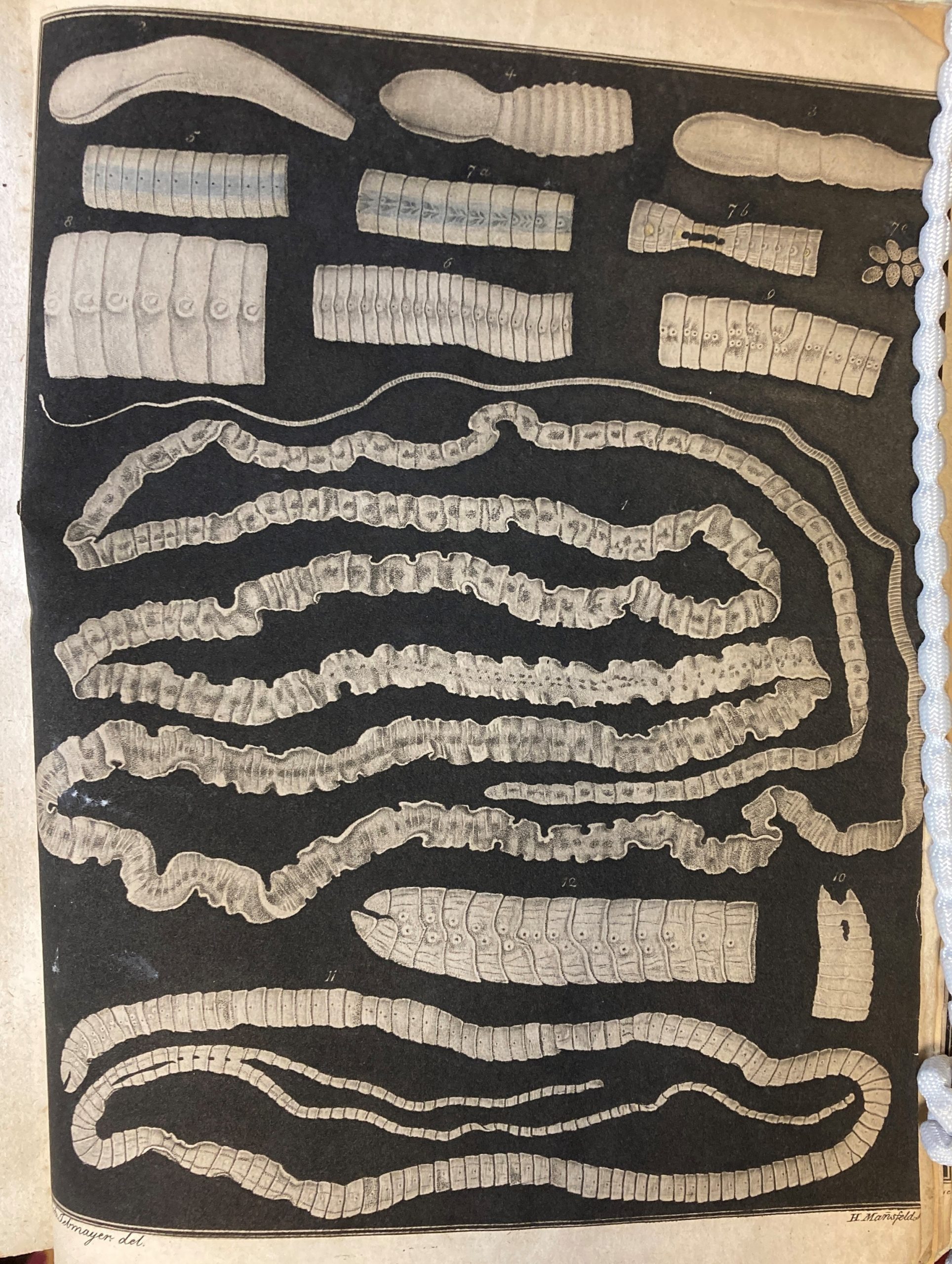This image appears to be a detailed page excerpt from a book or a museum catalog, likely showcasing various bones or fossils. The page is predominantly black, highlighting the white bones and fossils, which are intricately labeled with numbers such as 4, 3, 7, 6, 8, and 12 for identification. The specimens primarily consist of different vertebrae, resembling spinal cords, especially those depicted at the top of the page. A column of the bones extends thin and long through the middle, snaking across in a single, continuous line, with a similar structure mirrored at the bottom. The central section might depict dried snakeskin, while item 12 may resemble a talon or lobster claw. These anatomical drawings, attributed to H. Mansfield, suggest a focus on reptilian or amphibian skeletal structures, with snake skeletons prominently featured. The meticulous depiction and labeling of these specimens imply a detailed study or documentation of species, possibly for educational purposes.